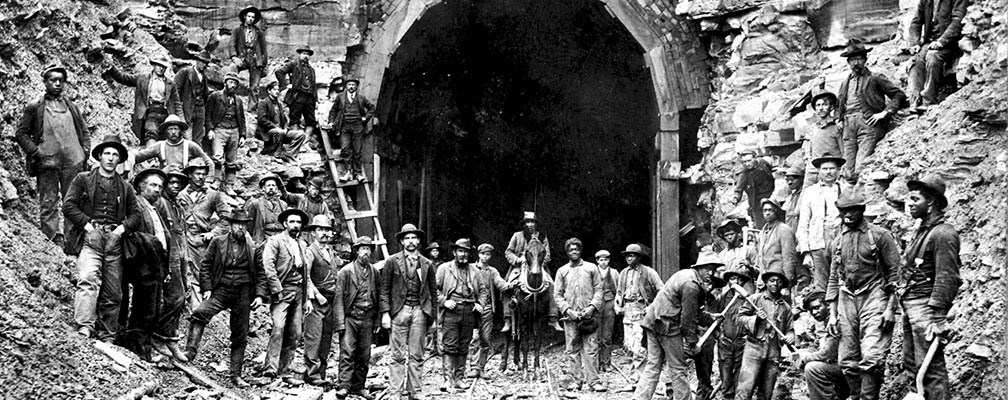A vintage black and white photograph captures an assembly of over 50 men standing around a large, curved tunnel entrance carved into a hillside or mountainside. The image is strikingly detailed, with men both on and around the tunnel, some standing at ground level and others positioned on cut-out portions of the rocky slope. In the center of the scene, a man is mounted on a dark horse, adding a focal point to the composition. The men's attire varies widely, ranging from shabby, laborer-like clothing to more formal business attire complete with suits and hats, painting a picture of a diverse group. On the left-hand side of the tunnel, a ladder extends upward with a man poised at its top. The rugged terrain surrounding the archway, with visible gravel and sand, further accentuates the vintage and historical feel of the photograph.